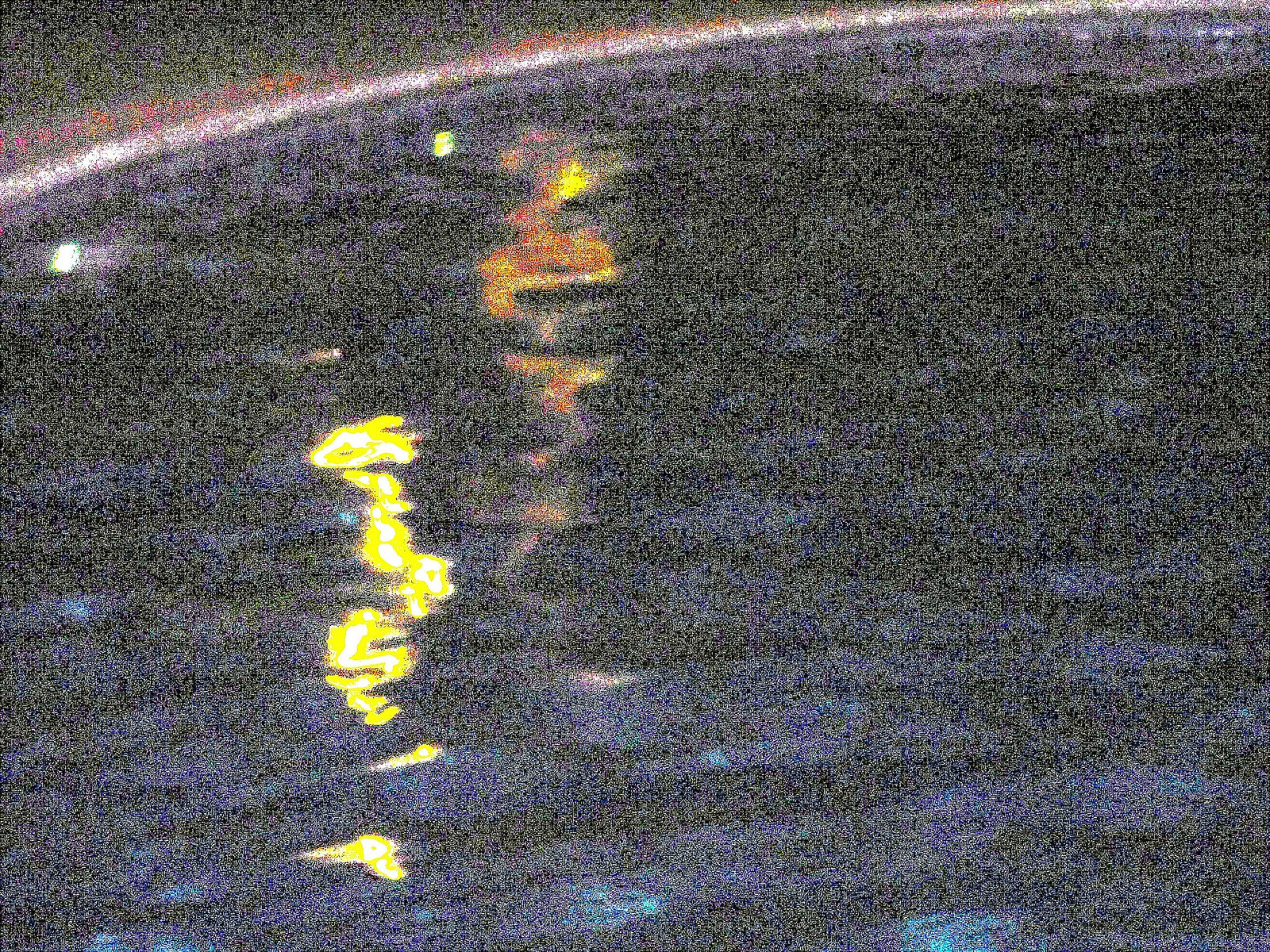This highly grainy and blurry image, resembling a poorly developed or corrupted digital photo, depicts what appears to be a home pool or hot tub. The photograph is dominated by blurred, abstract shapes and colors, implying water in motion. Notably, there are reflective elements, likely lights, creating yellow and orange blobs on the water's surface. Two key lights are visible inside the pool: a prominent one toward the center and another on the upper left. The top of the image features a recognizable rounded edge, suggesting a pool rim, while the upper left corner is entirely black. Despite the overwhelming graininess and overall fuzziness—evocative of television static—the image faintly portrays the rippling water's surface and faint light streaks, suggesting either a shining surface or fire lamps.